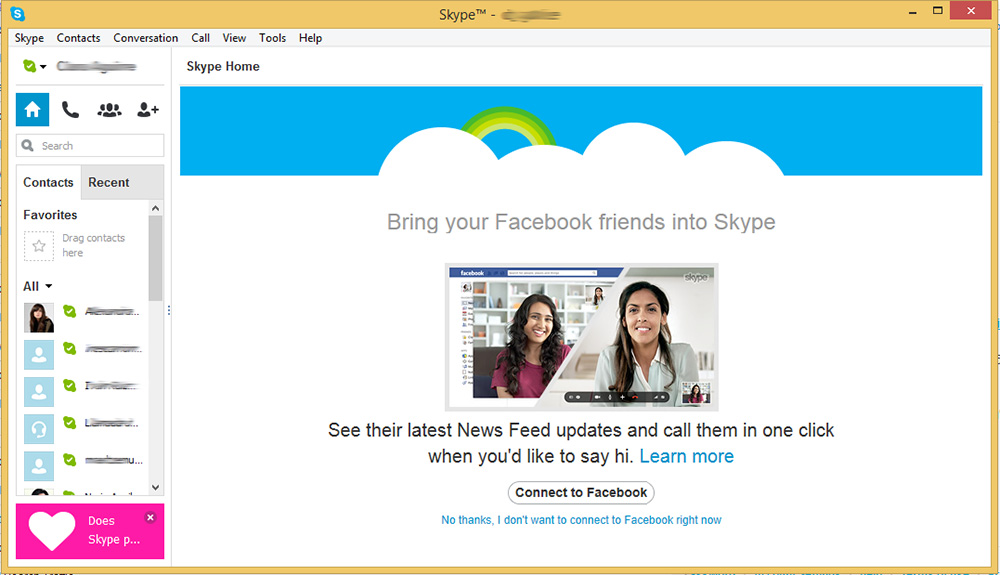In the image, we see a screenshot of the Skype application interface. Skype, a platform designed for video conferencing and online one-on-one interactions, utilizes a webcam for video communication on a computer. At the top of the screen, there's a distinctive orange bar displaying the title "Skype." On the right side of this bar, there's an "X" icon to close the application, a square icon to resize the window, and a minimize icon represented by a dash.

On the far left of the orange bar, there's the recognizable Skype logo, represented by an "S" encircled by a blue cloud. Below the bar, there's another taskbar featuring options such as Skype, Contacts, Conversation, Call, View, Tools, and Help.

Centrally positioned, there’s a promotional message encouraging users to integrate their Facebook account with Skype. The message reads: "Bring your Facebook friends into Skype," highlighting the ability to see the latest news feed updates and call them with one click. Beneath this message, there are two buttons: a blue "Learn More" button and a "Connect to Facebook" button. An additional option, “No Thanks,” is available for users who do not wish to connect their Facebook account at the moment.

The main section of the interface displays a split-screen video call between two women, indicating an ongoing interaction through Facebook on the top left corner. On the far left of the interface, there’s a blurred vertical toolbar. This toolbar includes icons for a check mark, home, call, group, and add a person features, followed by a search bar. Below the search bar is a contact list showcasing user contacts, along with their profile pictures if available. There's also a "Recent" tab and a heart icon, though the text next to the heart icon is cut off and not fully readable. Users have the option to exit this section if they prefer.